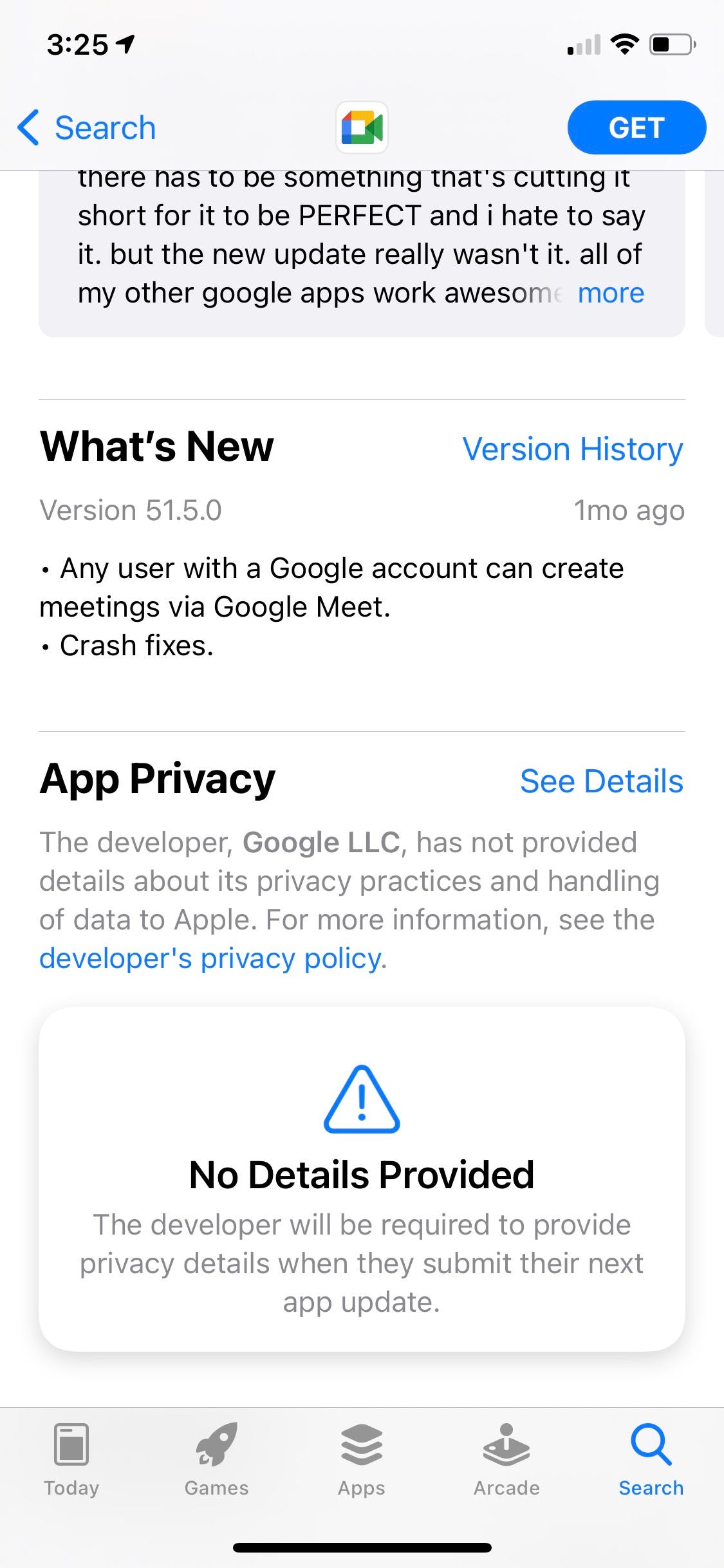The image is a screenshot taken from a smartphone. At the top of the screen, there is a grayish header. Below this header, the text "What's New" is prominently displayed. The background of the main content area is white. Moving further down, there is another white rectangle followed by a separate gray rectangle at the bottom of the screen.

The text at the top of the screen reads, "There has to be something that's cutting it short for it to be perfect and I hate to say it but the new update really wasn't it." This is followed by a comment on how all other Google Apps work well. Below this, there's a section that says, "What's New, Version History," along with the version number and a note indicating it was updated one month ago. This section mentions that "Any user with a Google account can create meetings via Google Meet," alongside "crash fixes."

Further down, it addresses app privacy, stating, "The developer Google LLC has not provided details about its privacy practices and handling of data to Apple. For more information see the developer's privacy policy."

Towards the bottom, a box has appeared with a blue exclamation point inside a triangle and the message, "No details provided. The developer will be required to provide privacy details when they submit their next app update."